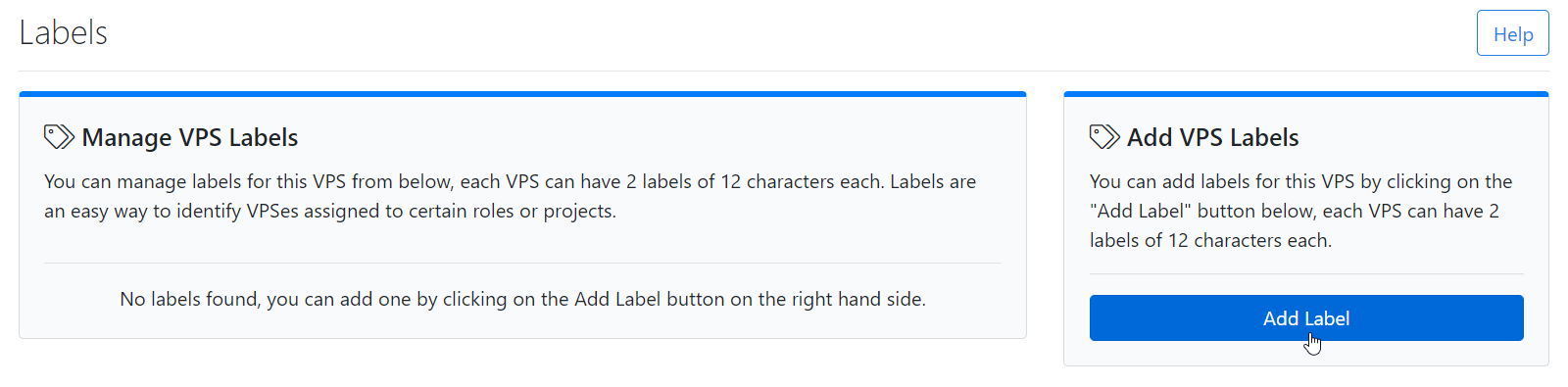This image showcases a sub-section of a troubleshooting or help page on a website, specifically focusing on VPS labels. The layout includes various elements neatly arranged for user guidance.

- **Top Left Corner**: The text "labels" is displayed.
- **Top Right Corner**: A button labeled "help" is available for additional assistance.

Below the header, there are two main sections:

1. **Manage VPS Labels Section**:
   - **Header**: A blue bar with the text "Manage VPS Labels."
   - **Description**: 
     - "You can manage VPS labels for this VPS from below. Each VPS can have two labels of 12 characters each. Labels are an easy way to identify VPS assigned to certain roles or projects."
   - **Status**: A note stating "No labels found."
   - **Instruction**: "You can add one or more by clicking on the add label button on the right side."

2. **Add VPS Labels Section**:
   - **Header**: Another blue bar titled "Add VPS Labels."
   - **Description**:
     - "You can add labels for this VPS by clicking on the add label button below. Each VPS can have two labels of 12 characters each."
   - **Action Button**: A prominent rectangular blue button labeled "Add Label."
   - **Mouse Pointer**: Positioned over the "Add Label" button, indicating a clickable action.

The overall background is white, and all the text is rendered in black for clear visibility. This structured layout ensures users can effectively manage and add VPS labels with ease.